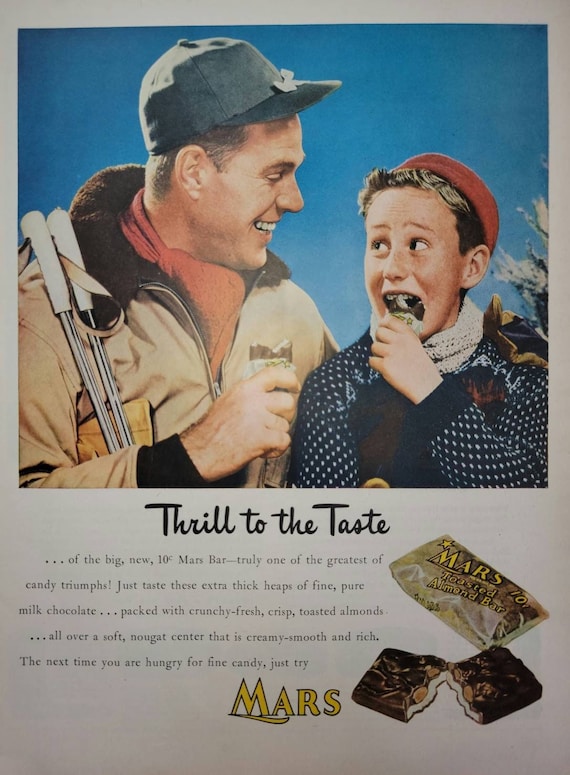In this vintage advertisement for Mars candy bars, a father and son are captured in a heartwarming moment as they enjoy chocolate bars together. Both figures are depicted in a style that blends photography with elements resembling a drawing. The son, dressed in a blue sweater with white checks and a red hat, looks excited while munching on his candy. The father complements the scene with his tan coat featuring brown fur trim and a blue baseball-style hat. Both are equipped with ski gear, including ski poles, and wear matching scarves, suggesting they might be on a skiing adventure.

At the center of the ad, the text invites viewers to "thrill to the taste of the big new 10 cent Mars bar, truly one of the greatest of candy triumphs." It describes the candy in mouth-watering detail: "extra thick heaps of fine pure milk chocolate packed with crunchy, fresh crisp toasted almonds all over a soft nougat center that is creamy, smooth and rich." 

To the right of this engaging description, there's a close-up shot of the Mars bar in its packaging, as well as an exposed view of a bar broken open to reveal its delectable interior. The overall color scheme of the advertisement features shades of blue, red, beige, and brown, set against a gray background, evoking a cozy, wintery feel perfect for the depicted skiing scenario.